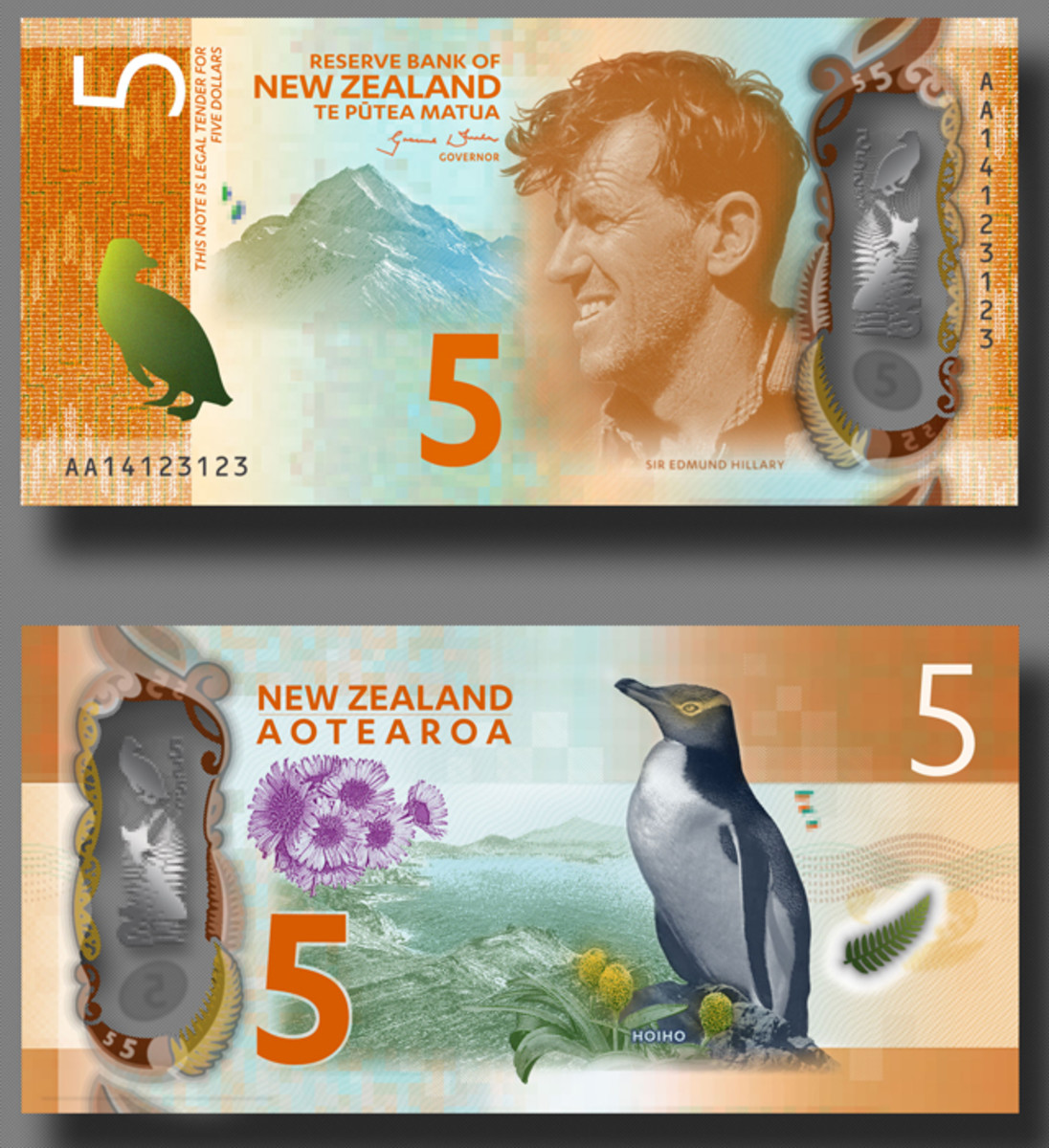This image shows two New Zealand five-dollar banknotes, positioned one above the other, against a dark gray background with subtle shadowing. The top banknote predominantly features an intricate design, with the text "Reserve Bank of New Zealand" displayed prominently. It showcases a green bird on the left side, a range of mountains in the center, and the face of Sir Edmund Hillary on the right side. Below the image of Sir Edmund Hillary, there is a serial number on the lower left, adding to its authenticity. The colors on this note include tones of reddish tan, with green and gray elements.

The bottom banknote also indicates a value of five dollars. It presents an engaging scene with a Hoi Ho (yellow-eyed penguin) depicted amidst a scenic background of the ocean, rocks, and purple flowers, which contrast with the penguin's distinct black and white plumage. Surrounding the penguin are additional details including green foliage. The text "New Zealand Aotearoa" is visible, adding cultural context. The primary colors on this note are orange with hints of green, blue, and purple in the center. Overall, the image provides a comprehensive view of these vibrantly designed pieces of currency, emphasizing their artistic and functional elements.